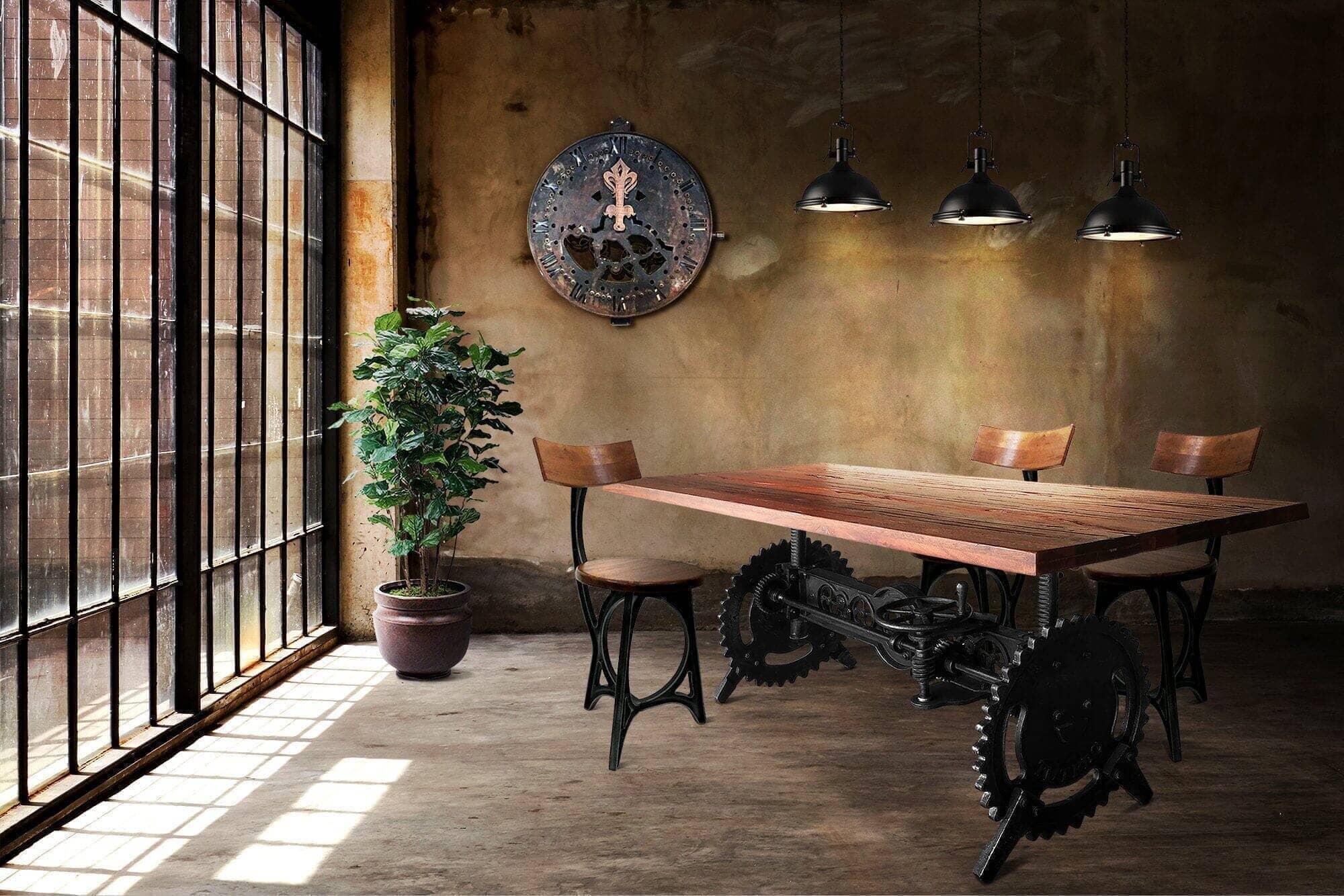The image depicts a moody, industrial-themed dining area, likely a coffee shop or bistro. On the left, a wall of tall, foggy and slightly dirty windows with a black and white wrought iron square pattern allows some light to filter in. Next to the windows stands a brown pot with a tall green plant, possibly artificial. The floor appears to be a lightly distressed hardwood with a brown marble coloration. The back wall, resembling unfinished warm tan concrete or rust-like paint, features a large artistic industrial metal clock with a copper hue. Central to the room is a wooden table with a darker brown top and an intricate base composed of large black gears and mechanical pieces, including a decorative crank. Around the table are three chairs with wooden backs and seats supported by black wrought iron frames, two facing the window and one facing them. Overhead, three black industrial-style lights hang down, casting regular white light onto the table below.